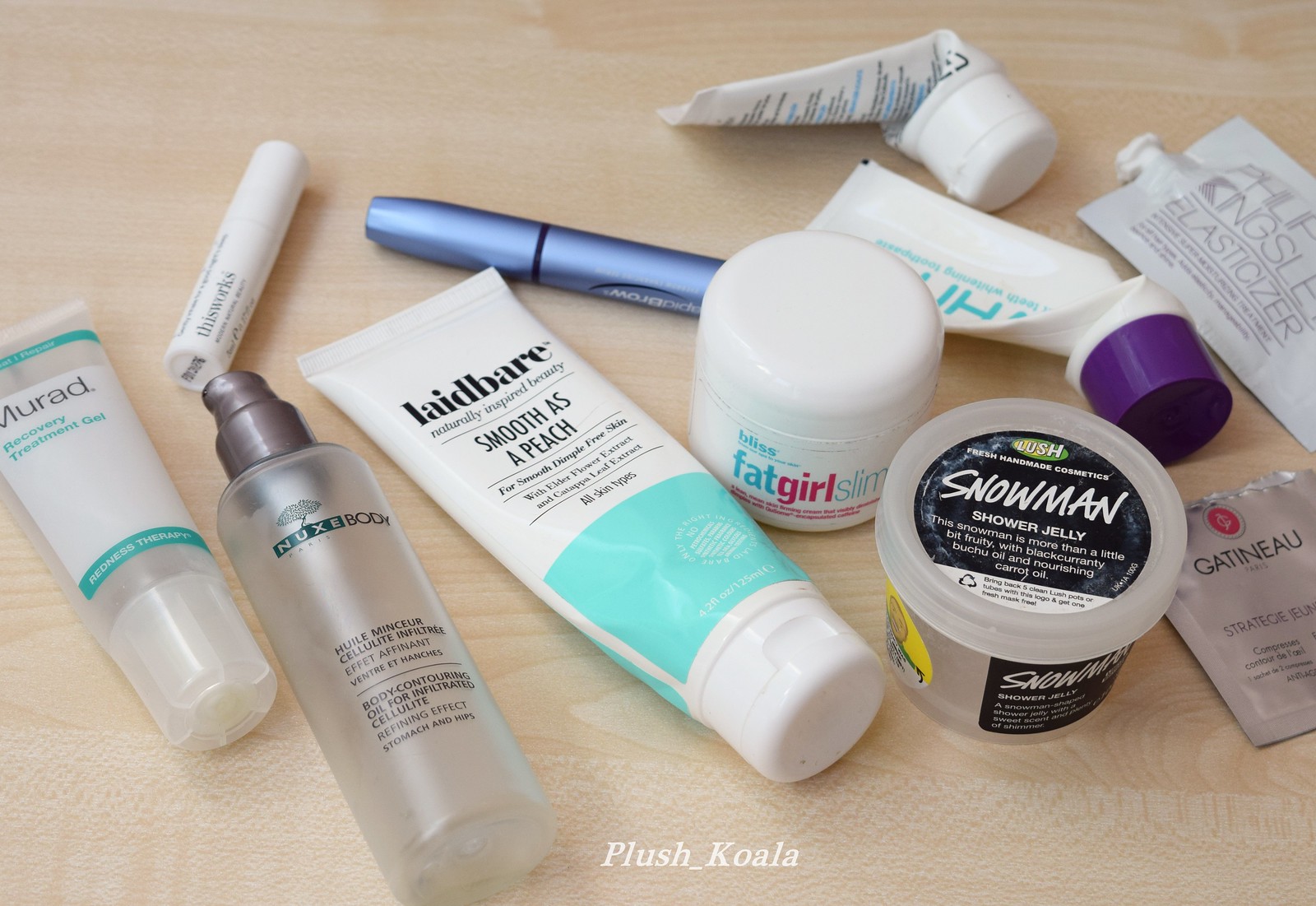This slightly overhead photograph captures an assortment of various sample-sized makeup products meticulously arranged on a light wooden surface. 

On the left, placed at an angle, is a clear squeeze container of Murad Recovery Treatment Gel. The gel has a distinctive rounded bottom, and the packaging features two teal lines at the top and bottom. "Murad" is printed in bold black, with "Recovery Treatment Gel" in matching teal font.

Moving right, there is a small, minimalist white tube with simple black text. This tube is angled towards the center of the photograph, lending a clean and sophisticated touch to the arrangement.

Next is a clear plastic bottle with an elegant, shiny brown pump top. It prominently displays "Nuxe Body" along with a tree logo, adding a touch of nature-inspired luxury to the scene.

At the center of the image, angled to the left, stands a small squeeze bottle with its lid at the bottom. This bottle carries the label "Laid Bare Smooth as a Peach," and features a blue banner across the bottom near the cap, promising a peachy smooth experience.

To the right of this bottle is a tiny white jar with a screw-off lid, boldly labeled "Fat Girl Slim." This jar adds a quirky and eye-catching element to the layout.

Continuing right, there is a small plastic container of Lush Snowman Shower Jelly. Its black label with white writing stands out, providing a festive hint against the other products. 

Behind this, towards the upper right, lies a completely exhausted tube with a rounded purple cap. Above it in the center area, another squeeze tube rests on its side, revealing only a partial view of the back label and a white flip-top cap at the bottom.

On the far right are two distinctive envelopes. One is a longer, aluminum packet with a squeeze top, prominently displaying the word "Elastidozer" in gold. Below this, angled to the left, is a smaller silver packet adorned with the words "Got No" in black, accompanied by a central red design.

Each product, from artisanal to clinical, is carefully positioned, creating a visually appealing and detailed representation of an exquisite range of beauty tools.